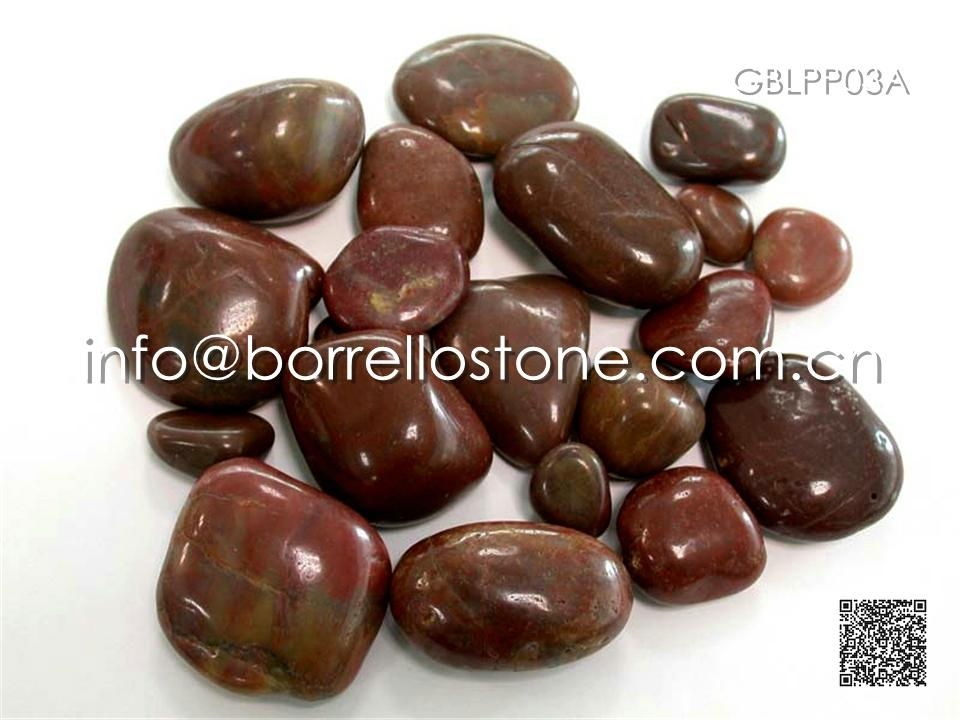The image reveals a collection of small, oblong, semi-polished stones in varying sizes that are mainly brown, with some exhibiting shades of reddish-brown and gray highlights. The stones are shiny and appear to be carefully arranged, with some overlapping and others spread out on a white background. Centered in the image is an email address, "info@borellostone.com.cm," and in the upper right corner, there is a text string in uppercase, "GBLPP03A." Additionally, a scannable QR code is located in the bottom right corner. The camera angle is slightly elevated and zoomed in, providing a detailed close-up of the stones, which might be intended for jewelry or rock collection advertisement.